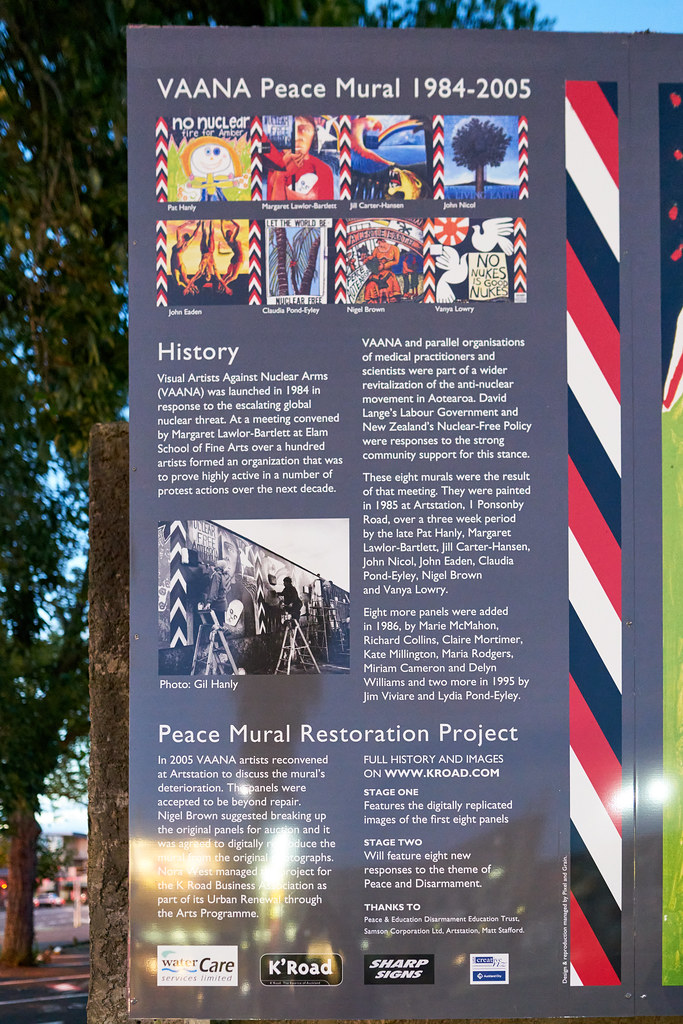The image features a detailed vertical banner titled "Vanna Peace Mural 1984-2005" at the top. The banner has various illustrations, including stick figures, cartoon characters, trees, birds, and other abstract art arranged in rows. In addition to these colorful drawings, there are black-and-white photographs depicting people painting murals. In the middle section, the text "Peace Mural Restoration Project" is prominently displayed alongside detailed historical information in paragraphs. At the bottom of the banner are four distinct logos, including Water Care, K Road, Sharp Signs, and another partly obscured one. The right side of the banner displays red, white, and black stripes. In the background, vibrant green trees, a fragment of a street, and a blurred car indicate that the setting is sunny and outdoors.